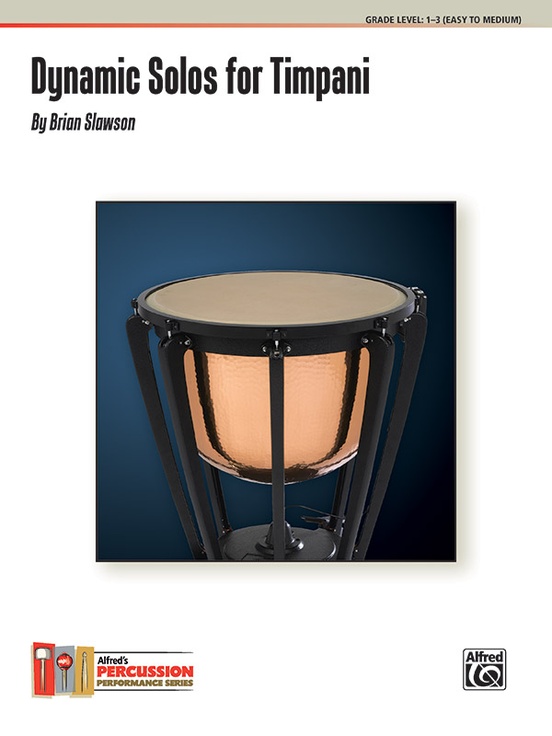This is a color photo of a book cover for "Dynamic Solos for Timpani" by Brian Slauson, featured as part of Alfred's Percussion Performance Series. The cover prominently displays text at the top that reads "Grade Level 1 to 3, Easy to Medium" and "Dynamic Solos for Timpani by Brian Slauson." The main image is of a timpani drum, which is black with vertical lines and has a copper or metallic bottom part. The drum is set against a dark blue background. At the bottom left of the cover, the text "Alfred's Percussion Performance Series" is accompanied by three illustrated drumsticks. In the bottom right corner, there is an Alfred logo with a treble clef design inside a square. The overall quality of the image is good, and the text is written clearly in black.